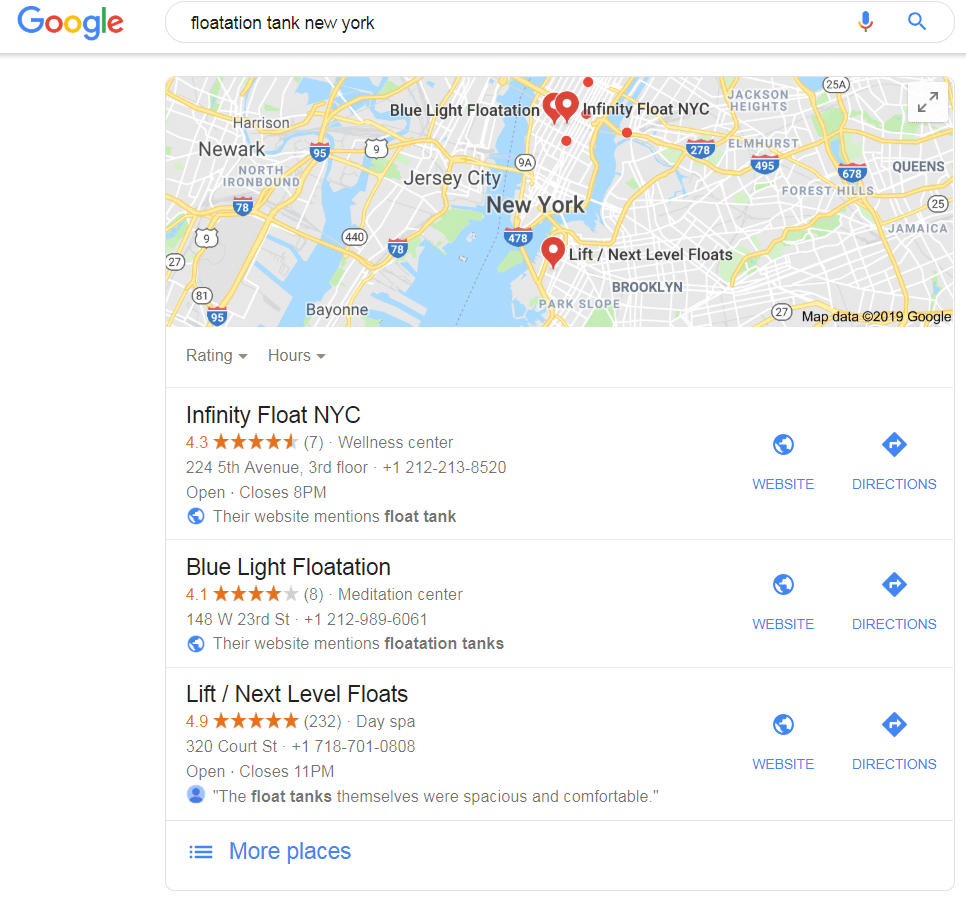The image displays a Google search results page for "flotation tank New York." At the top, within the search bar, is the text "flotation tank New York," accompanied by the microphone icon and the search button.

In the search results, the map indicates locations within New York, including notable areas like Newark. Below the map, sections are labeled "Rating and Hours."

1. The first listing is for "Infinity Float NYC," rated 4.3 stars from 7 reviews, categorized under "Wellness Center." The address is 224 5th Avenue, 3rd Floor. The listing notes that the center opens and closes at 8 PM, has a website mentioning float tanks, and offers buttons for both their website and directions.
   
2. The second entry is "Blue Light Flotation," rated 4.1 stars, categorized under "Meditation Center." This listing includes the address and indicates that the website mentions flotation tanks. There are buttons for the website and directions displayed to the right in blue.
   
3. The third listing is "Lift/Next Level Floats," with a high rating of 4.9 stars from 232 reviews, categorized under "Day Spa." It provides the option for both the website and directions, noting that it closes at 11 PM. 

At the bottom of the image, there is an option labeled "More places," suggesting additional listings can be viewed.